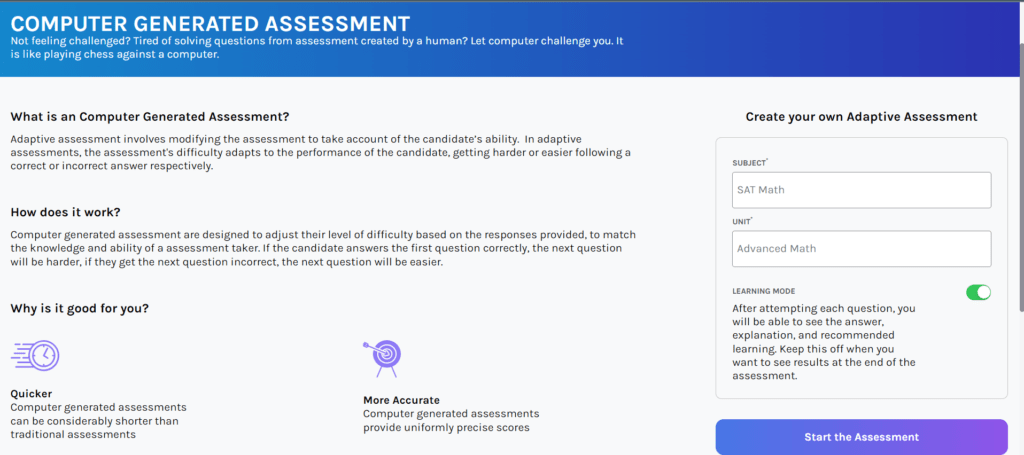The image depicts an interface with a light gray background and a prominent thick blue bar at the top displaying the heading "COMPUTER GENERATED ASSESSMENT" in white uppercase letters. Below this heading, white text reads, "Not Feeling Challenged, Tired of Solving Questions from Assessment Created by a Human, Let Computer Challenge You. It is like playing chess against a computer."

On the right side, a black header reads, "Create Your Own Adaptive Assessment." Beneath this header is a square outlined with a thin gray line, containing two text entry boxes. The first box, labeled "Subject," has "SAT Math" typed in, while the second box, labeled "Unit," has "Advanced Math" typed in. Below these boxes, the text "Learning Mode" is displayed next to a toggle button that is switched on. Further down, a blue button labeled "Start the Assessment" is visible.

To the right of the text entry area, there is additional text accompanied by a couple of icons. The layout suggests a comprehensive and user-friendly interface designed for creating personalized, computer-generated assessments.